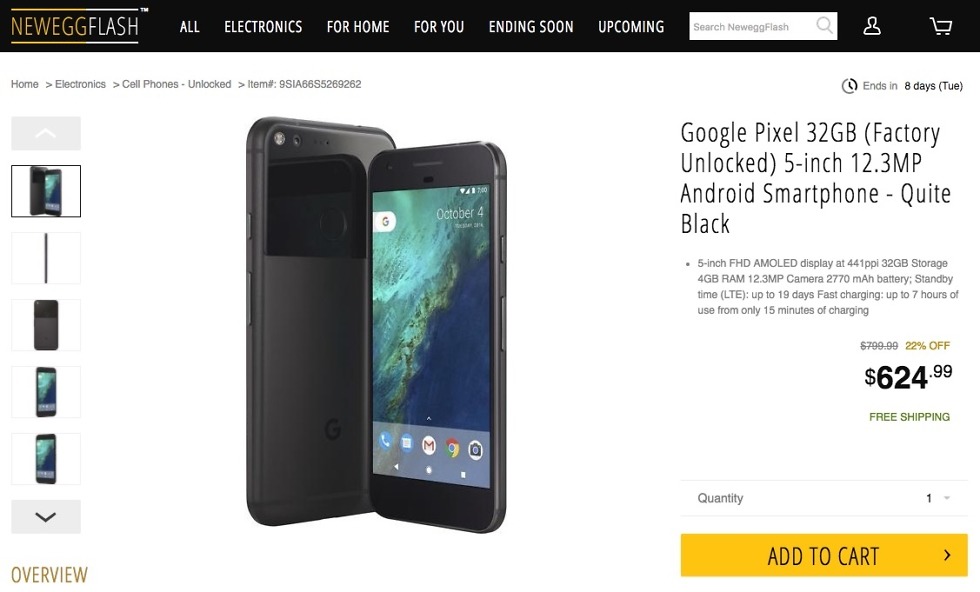**Screenshot from Newegg Flash Product Page Featuring Google Pixel Smartphone**

The image is a detailed screenshot of a product page on the Newegg Flash website. At the top left corner, the Newegg Flash logo is prominently displayed, indicating the online platform for flash deals. Below the logo, multiple categories are listed in a horizontal menu bar, including "All," "Electronics," "For Home," "For You," "Ending Soon," and "Upcoming."

Centered in the middle of the page is a high-resolution image showcasing the front and back of a sleek smartphone. To the right of the image, the product details are clearly listed: 
"Google Pixel 32 GB Factory Unlocked 5-Inch 12.3 MP Android Smartphone, Quite Black." 

The product's brief description further highlights its key feature, boasting a "5-Inch FHD Display." 

At the bottom, the price is prominently displayed in bold text: "$624.99."

The layout is clean and visually appealing, focused on providing essential information at a glance.